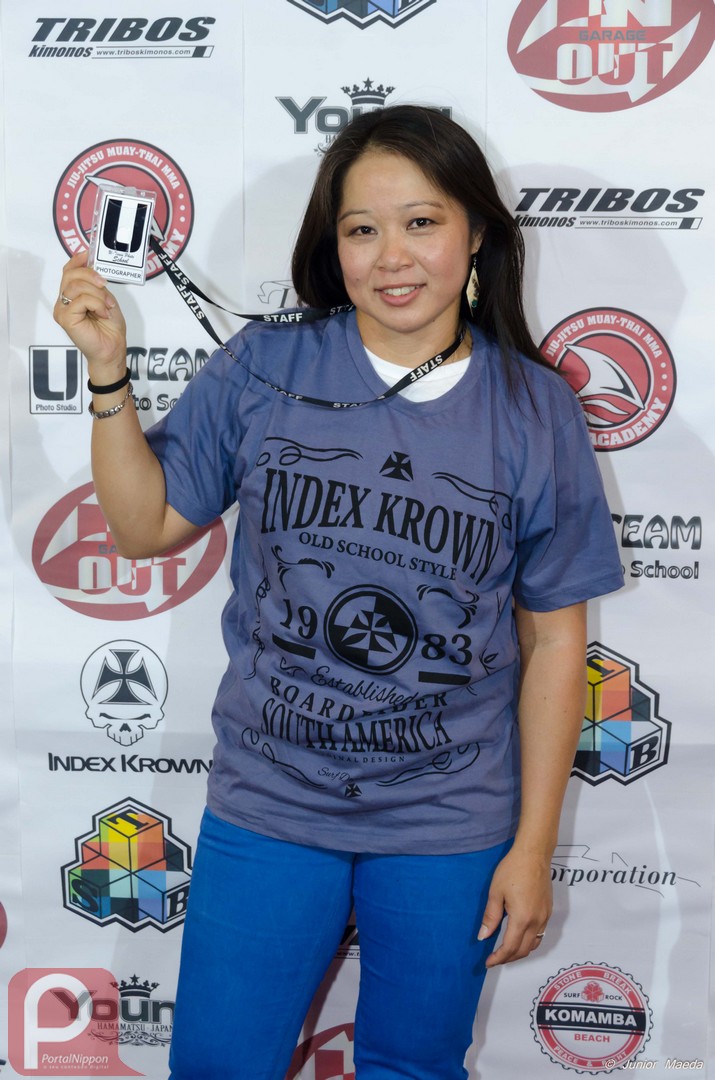In this full-color photograph, a young Asian woman with long brown hair stands against a white-gray background filled with various sponsor logos, including Index Crown (spelled with a K), Kamamba, and Tribose. She is dressed in a purple-blue shirt with black text that says "Index Krown," along with the year "1983" in an old-school style. Beneath the text are additional details, including the words "South America" amidst a circular design featuring an old German cross in a purple and black style. Under her shirt, she wears a white t-shirt, and she has dark blue pants. Around her neck, she wears a black lanyard from which a placard hangs, displaying a large letter "U." She's holding up the placard with her right hand, which also sports a black wristband and a silver bracelet, while her left hand hangs by her side. The setting appears to be indoors.